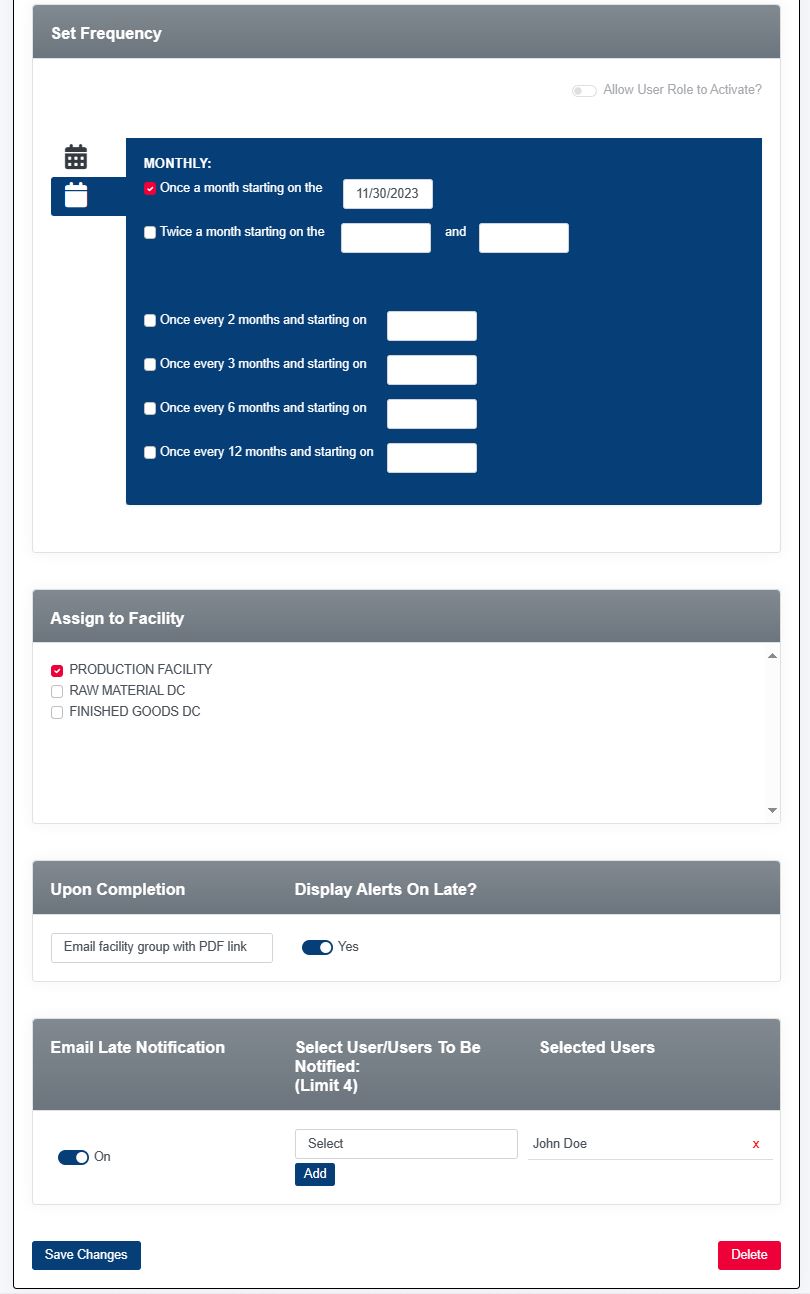*Screenshot Description:*

The screenshot features a detailed interface for setting frequency schedules and assigning facilities, along with notification preferences.

- **Set Frequency Section:**
  - **Top Border:** Gray with white text on the left stating "Set Frequency."
  - **Left Side:** Gray text that asks, "Allow user role to activate?" followed by a question mark.
  - **Main Body:** White background.
  - **Frequency Options:**
    - A blue rectangle with white text stating "Monthly... Once a month starting on 11-30-23."
    - "Twice a month on" followed by two empty boxes for customization.
    - "Once every two months starting on," followed by an empty box.
    - "Once every three months starting on," followed by an empty box.
    - "Once every six months starting on," followed by an empty box.
    - "Once every 12 months starting on," followed by an empty box.
  - **Selection Column:** On the left side of each frequency option, there is a checkbox. The first checkbox is selected, which is indicated by a red box with a white check mark.

- **Assign Facility Section:**
  - **Separator:** A gray line and border.
  - **Header:** White text on a gray background stating "Assign Facility."
  - **Facility Options (in black text with white background):**
    - "Production Facility"
    - "Raw Materials DC"
    - "Finished Goods DC"
  - **Selection Column:** Each option has a checkbox next to it. The first checkbox is selected, indicated by a red box with a white check mark.

- **Upon Completion Section:**
  - **Separator:** A gray banner.
  - **Header:** White text on a gray background stating "Upon Completion."
  - **Options (in black text on white background):**
    - "Display alerts on late?" followed by a question mark.
    - "Email facility group with PDF link." The response indicated is "Yes."
    - "Email late notifications?"
    - "Select user/users to be notified, limit four." Options to select users are provided.

This detailed interface allows users to specify scheduling intervals, assign facilities, and set up completion notifications effectively.